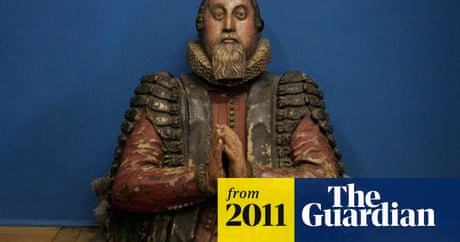The image captures a highly detailed, vintage sculpture of a man in front of a blue wall. The man has a neatly trimmed brown beard and brown hair. He is dressed in black armor with horizontal straps on the sleeves and an elaborate red robe underneath. Around his neck, he bears a distinctive ruffled collar, giving a nod to his noble status. His hands are clasped together in a praying position, adding an element of solemnity. The photograph of this weathered artifact is clear and brightly lit, enhancing every intricate feature of the sculpture. In the bottom right corner, there are two rectangles: one yellow with the text "from 2011" and one dark navy blue with the text "the Guardian" in white, indicating the image's source.